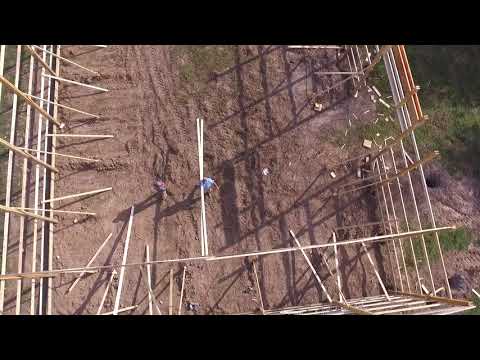An aerial, top-down view of a construction site reveals the skeletal frame of a rectangular or square structure, primarily composed of light-colored wood arranged both vertically and horizontally. Despite the overall low resolution of the image, certain details stand out: the frame is predominantly visible along the left side and the bottom right corner, with a possible entrance or exit appearing as a break in the wooden structure near the top right. Inside the structure, the ground is rough and brown, indicative of dirt, with sparse patches of green grass visible around the perimeter.

Inside the framework, two individuals can be seen. One, placed centrally, is identifiable by a blue shirt and carries two long planks of wood, with additional details such as his left arm being raised. The second individual, wearing a brownish shirt, is less detailed but discernible. Alongside the main structural beams, numerous light-colored sticks and supporting beams are seen leaning against and balanced within the framework. The surrounding area outside the structure features a mix of brown dirt and small grassy patches, hinting at early-stage construction and groundwork.